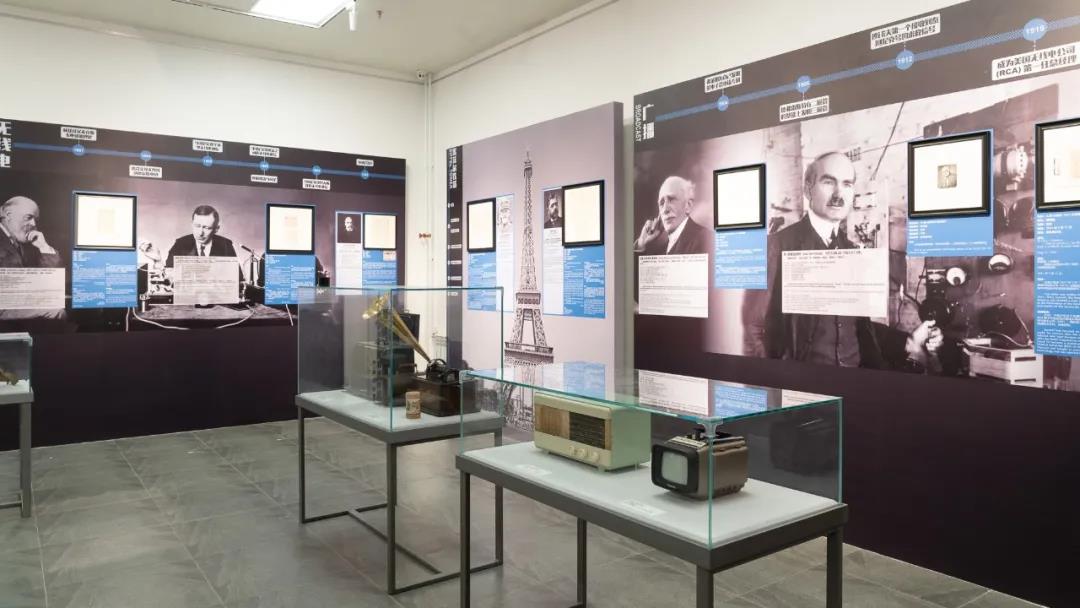The photograph depicts the interior of a museum room with white walls, a gray patterned floor, and a white ceiling featuring fluorescent lighting. The walls are adorned with large blue informational boards that outline timelines, paragraphs of text, and black and white photographs of various inventors and historical figures. Several glass display cases are situated on tables supported by metal bars, each containing vintage electronic equipment and artifacts. Notable items include a beige rectangular device with three circular knobs and a digital screen, and a brown square object resembling an old television encased in another display. Additionally, one case showcases an artifact similar to a jukebox with a prominent gold megaphone, and another potentially houses an early radio. The overall scene is carefully organized, blending historical information with tangible exhibits to create an educational atmosphere.